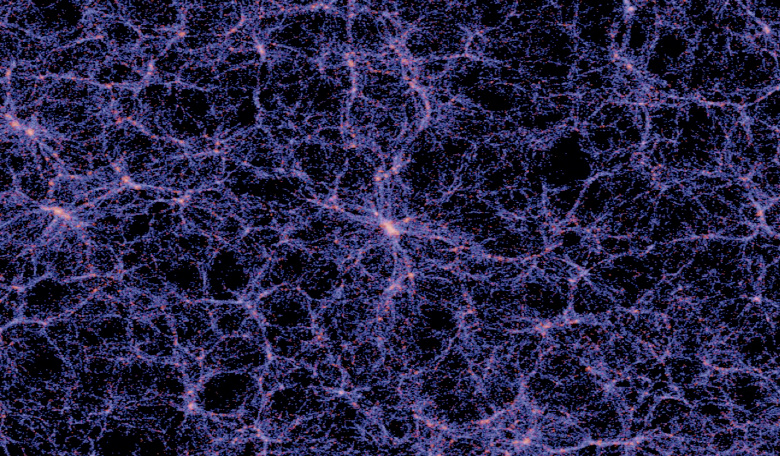The image showcases an intricate, almost microscopic close-up that immerses the viewer in a tapestry of dark, deep hues dominated by black and purple, accented with a scattering of orange and red tones. It resembles a highly detailed fibrous carpet or static electricity, with numerous fine strands and webs weaving across the frame. This elaborate network suggests a scientific visualization possibly akin to nerve endings or the scattered patterns of static on a television screen, but with much more depth and complexity. The dark background is punctuated by grayish-purple fuzz and occasional bright clusters, highlighting centers of white and red. Particularly in the middle, the texture brightens with hints of orange and red, creating a focal point amid the endless, chaotic yet captivating web of predominantly purple strands. This image, laden with a sense of static electricity and random, spider web-like distributions, conjures an almost alien yet scientifically fascinating visual experience.